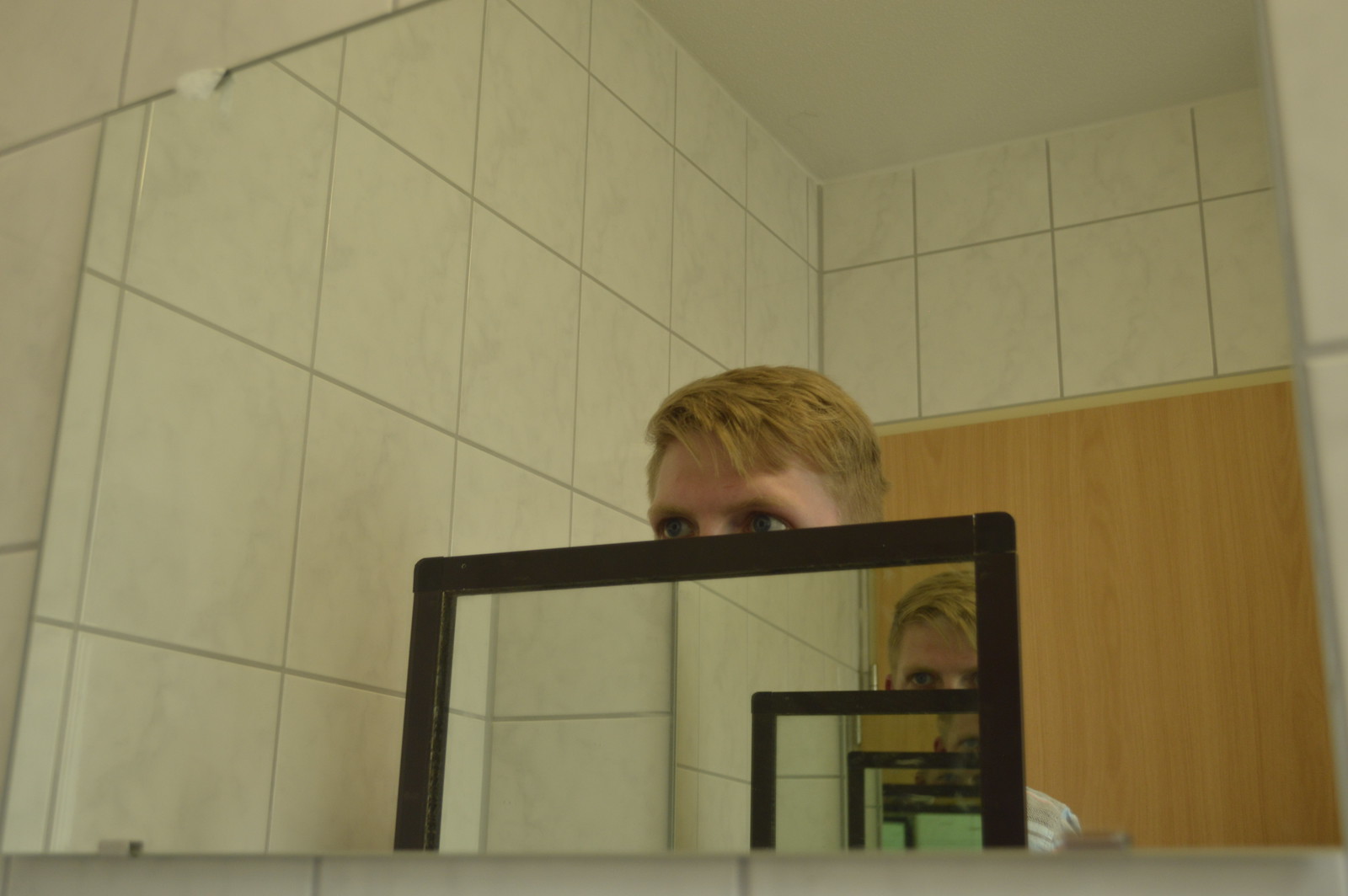In this color photograph taken indoors in landscape mode, a man is standing in front of a rectangular, horizontal bathroom mirror, partially obscured by a smaller, dark-framed mirror he holds up. The room, which resembles a cubicle or shower stall, features large, light beige tiled walls, a wooden door, and a white ceiling. The man's pale complexion, short light auburn hair, and dark eyebrows are clearly visible, as are his wide, intently staring eyes. Due to the smaller mirror he holds in front of his face, we see a cascading "infinity effect" within the large mirror's reflection, creating the illusion of the man's face and the frame repeating three times toward the lower right.